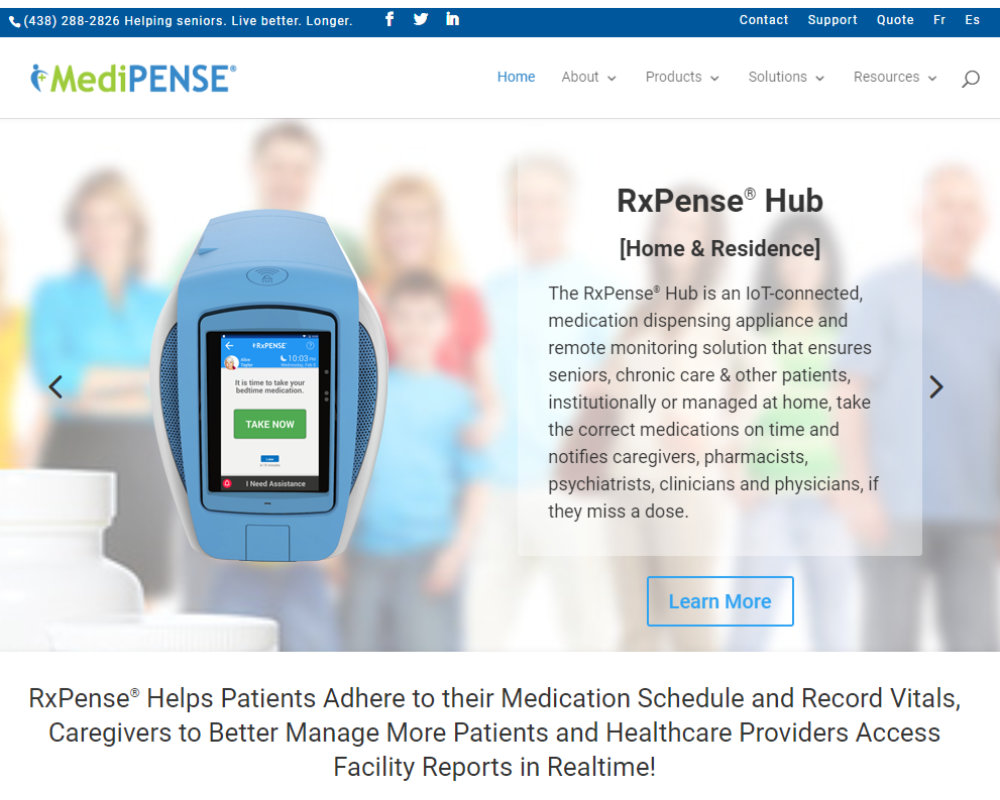In this screenshot of the MediPens website, the upper left corner prominently displays the company's phone number, 438-288-2826, alongside the slogan "Helping seniors live better, longer." On the upper right corner, a prompt reads "Contact support: FRES," indicating a support service option. The navigation bar at the top contains multiple tabs including Home, About, Products, Solutions, Resources, and a Search bar, with the current view set to the Home tab. 

Central to the page is an image of the MediPens device, accompanied by a pop-up box detailing its features. The device, named RxPensHub, is described as an IoT-connected medication dispensing appliance geared towards home and residential use. This system aims to help seniors, individuals under chronic care, and other patients manage their medications accurately at home. The solution includes remote monitoring capabilities, notifying caregivers, pharmacists, psychiatrists, clinicians, and physicians if a dose is missed, ensuring comprehensive care management. 

Beneath this detailed description is a blue outline rectangle featuring the text "Learn more," inviting users to explore further information about the RxPensHub and its benefits.